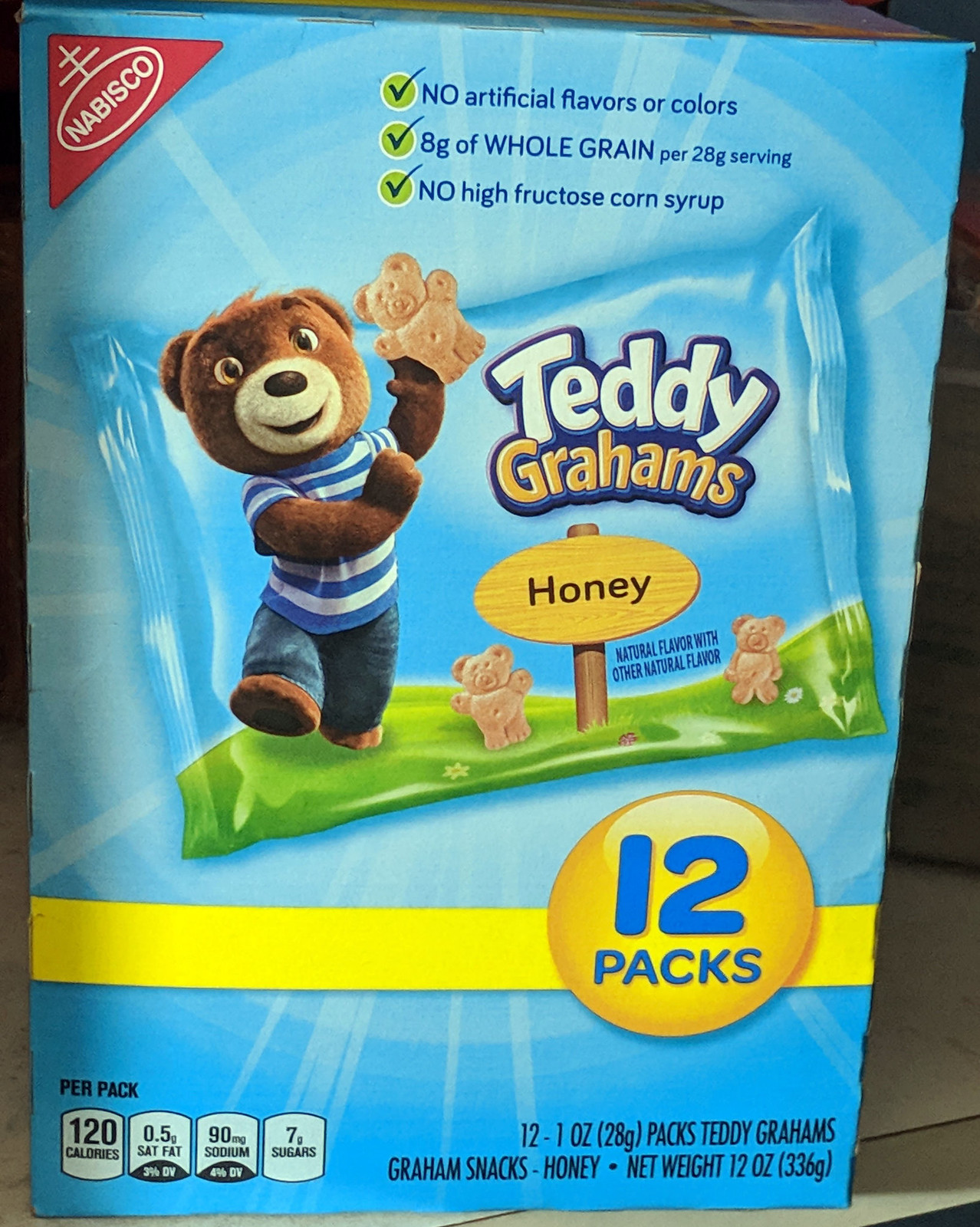This is a photograph of a blue cardboard box of Nabisco Teddy Grahams, emphasizing its honey flavor. The box, prominently displaying the Nabisco logo—a red triangle with a white circle in the corner—contains 12 individual 1-ounce (28-gram) packs, amounting to a total net weight of 12 ounces (336 grams). The packaging features a dark brown, cartoon bear character wearing a blue and white striped shirt and blue pants, holding a Teddy Graham cookie. Two additional cookies lie on the ground beside the bear. The box highlights several health claims in green circles with blue check marks, stating "No Artificial Flavors or Colors," "8 grams of Whole Grain per 28 gram serving," and "No High Fructose Corn Syrup." Nutritional information at the bottom notes each pack contains 120 calories, 0.5 grams of saturated fat, 90 milligrams of sodium, and 7 grams of sugar. The background contrasts with a white countertop, accentuating the box’s details, including the product name "Teddy Grahams," with "Teddy" in white and "Grahams" in gold letters.